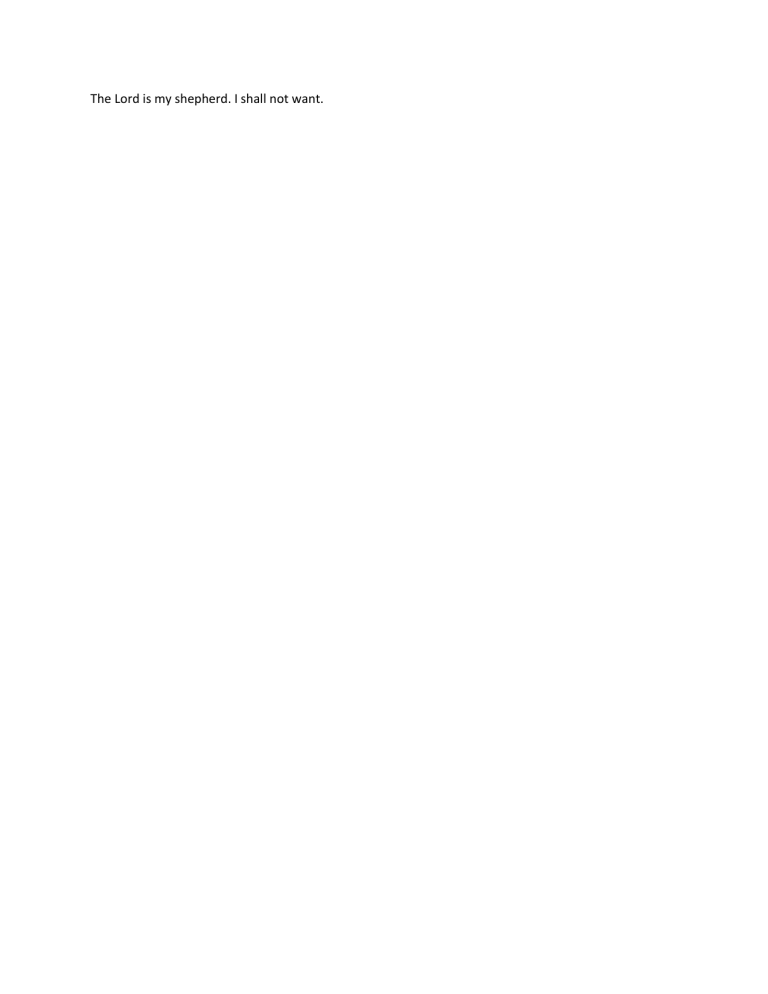The image depicts a minimalist composition with an entirely white background, which seamlessly merges with the color of an empty computer screen. Amidst this stark expanse, the only discernible element is a line of very small black text, likely in 6-point Arial or another sans-serif font. The text reads: "The Lord is my shepherd. I shall not want." This snippet is a recognizable excerpt from a psalm in the Bible. Each initial letter of the two sentences is capitalized, adhering to proper grammatical standards. There are no additional markings, notations, or references such as chapter and verse numbers accompanying the text. The simplicity of the image highlights the text's spiritual message without any distractions, as there are no borders, outlines, or surrounding elements to detract from the words.